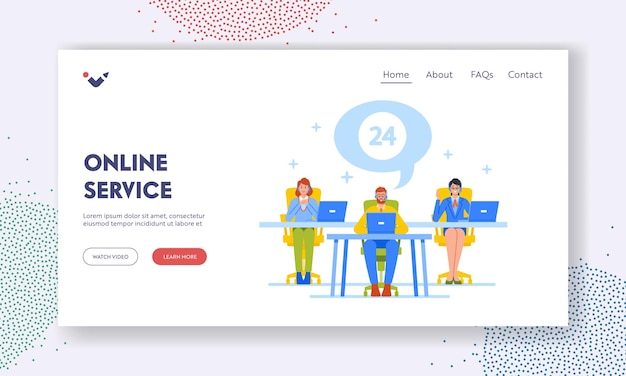This image depicts the front page of a website or app interface. The background is predominantly off-white with several colored dot patterns: a blue circle of dots in the bottom right, a green circle in the bottom left, and a red circle in the upper left. Central to the image is a rectangular section outlined by a colorful border. Along the top of this section is a navigation menu displaying the options "Home," "About," "FAQs," and "Contact." 

Below the menu, three cartoon-style illustrations of people (two women and one man) are sitting at desks with laptops. A large blue speech bubble with a "24" in it hovers over their heads. To the left of these characters, large text reads "Online Service" followed by placeholder text: "Lorem Ipsum, Dottor Set Aman Consecutor Estus Ius Tempor Incident Ut Labora Et." Additional elements include a white button and a red toggle button beside the text. At the bottom, there are options to "Watch video" or "Learn more."